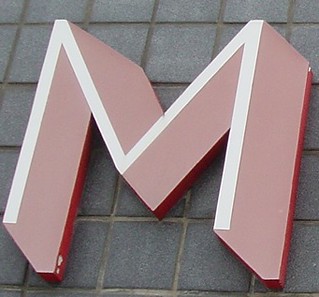The image prominently features a large, three-dimensional letter "M" that takes up most of the frame, creating a stark and bold visual impact. The background is composed of gray cinder block squares, each delineated by light brown or tan grout. The squares are arranged in a grid pattern, with some blocks showing more dirt and wear at the top compared to those at the bottom.

The "M" itself stands out dramatically from the wall, projecting outward by about a foot. The base of the letter is red, with noticeable scuff marks that reveal white patches underneath. The sides of the "M" are a gradient of pinkish white, adding dimensionality further accentuated by shadows that suggest a strong light source. The top and front face of the "M" are stark white, with the letter’s structure featuring sharp, angular points that meet at the center, creating a striking contrast against the rough gray backdrop.